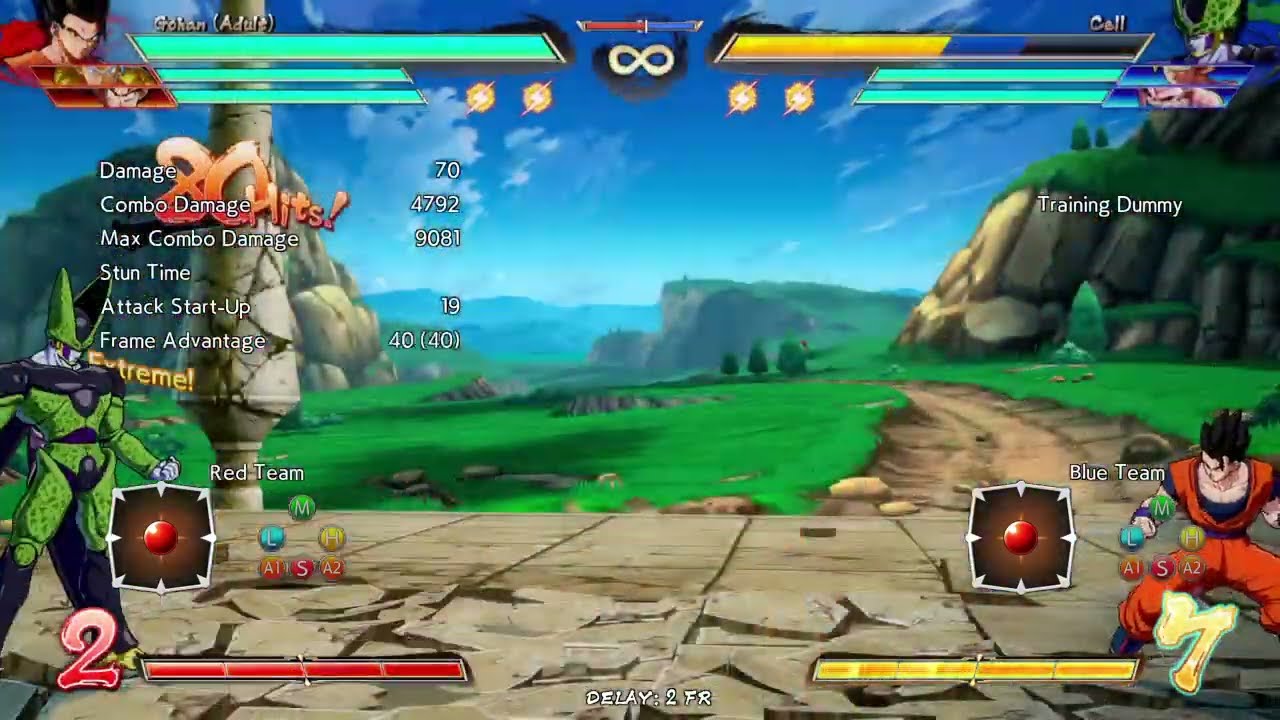The image is a high-definition screenshot from the Dragon Ball Z video game, depicting an intense combat scene. In the foreground, two characters face off on a stone platform amid a lush green grassland with mountains in the background under a clear blue sky. On the bottom right is Gohan, clad in an orange muscle shirt and pants with black spiky hair, appearing muscular and ready for battle. On the bottom left is Cell, a character with white skin, green body armor, and a tall head with two pointy parts. The interface shows player stats, with Gohan having a score of seven (displayed in yellow) and Cell with a score of two (displayed in red). Additionally, there is a sidebar with detailed combat metrics including damage and combo damage. The scene captures a dynamic moment in a combat video game, emphasizing the vibrant backdrop and the tension between the two fighters.